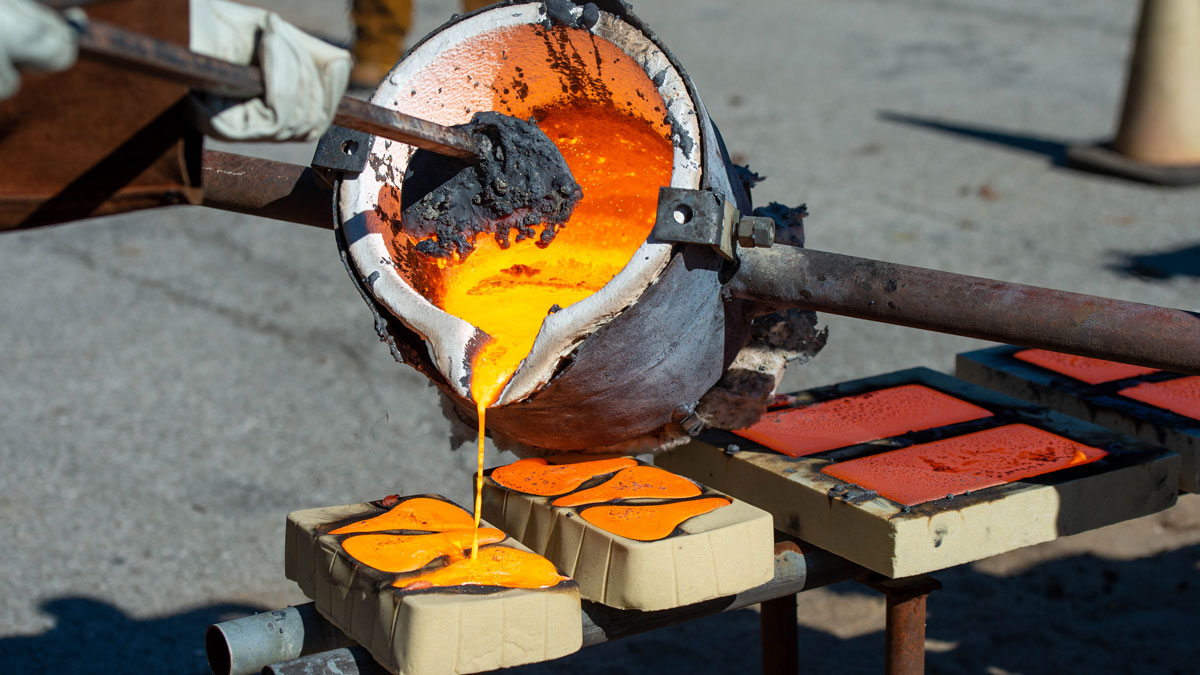In this photograph, a metal smelter is in the process of pouring molten metal into various molds. The glowing, red-hot metal, which appears to be steel, is being carefully managed from a large metal bucket with a white ceramic lining and a spout for pouring. In the foreground, a person's hands are visible, covered with thick white gloves and encased in thick brown leather sleeves, indicating protective gear against the heat. They grip a long, rusty brown spade-like tool with a semicircular head, encrusted with slag and metal, which they use to manipulate and guide the molten metal. The person is operating the spout to pour the yellow-orange, liquified steel into tan-colored molds. These molds are rectangular, resembling bricks, and there is also a distinct pear-shaped mold evident in the scene. The pouring process is meticulously controlled, showcasing the intense, glowing metal transitioning into solid forms.